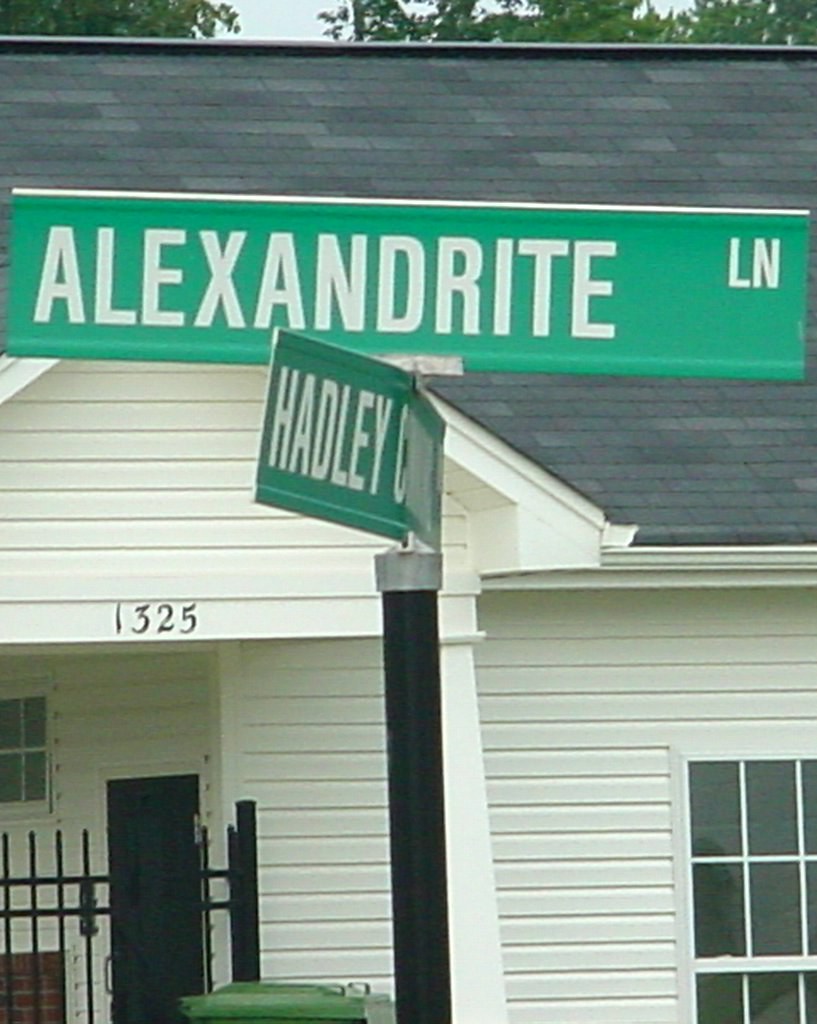The photograph captures an outdoor scene centered around two intersecting street signs on a black pole with a silver cap. The top green sign, labeled "Alexandrite LN" in white letters, sits perpendicular to another green sign below it, which seems to read "Hadley" but is partially obscured due to its angled positioning. The setting includes a white house with white siding and pillars, featuring a black front door and a window with a white wood divider on the left side. The house roof is clad in black shingles, and a house number "1325" is visible on a timber beam across the portico. A black metal gate secures the entryway. Adjacent to the house is the edge of a red brick wall with dark gray grout. The scene is framed by dark green leafy trees under an overcast sky with shades of blue and gray. In the foreground, near the pole, is a green trash can.